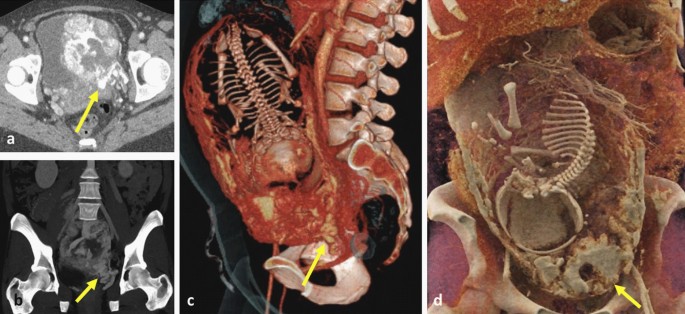The image presents a set of four distinct medical images labeled A, B, C, and D, showcasing various anatomy slides utilizing different imaging techniques. Slides A and B, positioned one above the other on the left side, are both black and white with prominent yellow arrows highlighting specific anatomical features. Slide A appears to be a traditional ultrasound image, while Slide B resembles an enhanced x-ray, possibly augmented with illustrative highlights of body parts.

Slide C, located in the center, is a vivid and colorful depiction of a cadaver, possibly prepared with plasticine and dissected to reveal internal structures. The remarkable detail reveals a pregnant woman, observable by the presence of two spines—one large and one small. Slide D, similar in size and placement to Slide C but on the right side, continues with the theme of colorful anatomical dissections, focusing on a region around the spine and hips. This slide is resplendent with red, white, and purple hues, detailing the spinal column, hip bones, and possibly other organs within the ribcage area, again marked by a yellow arrow pointing to a specific structure.